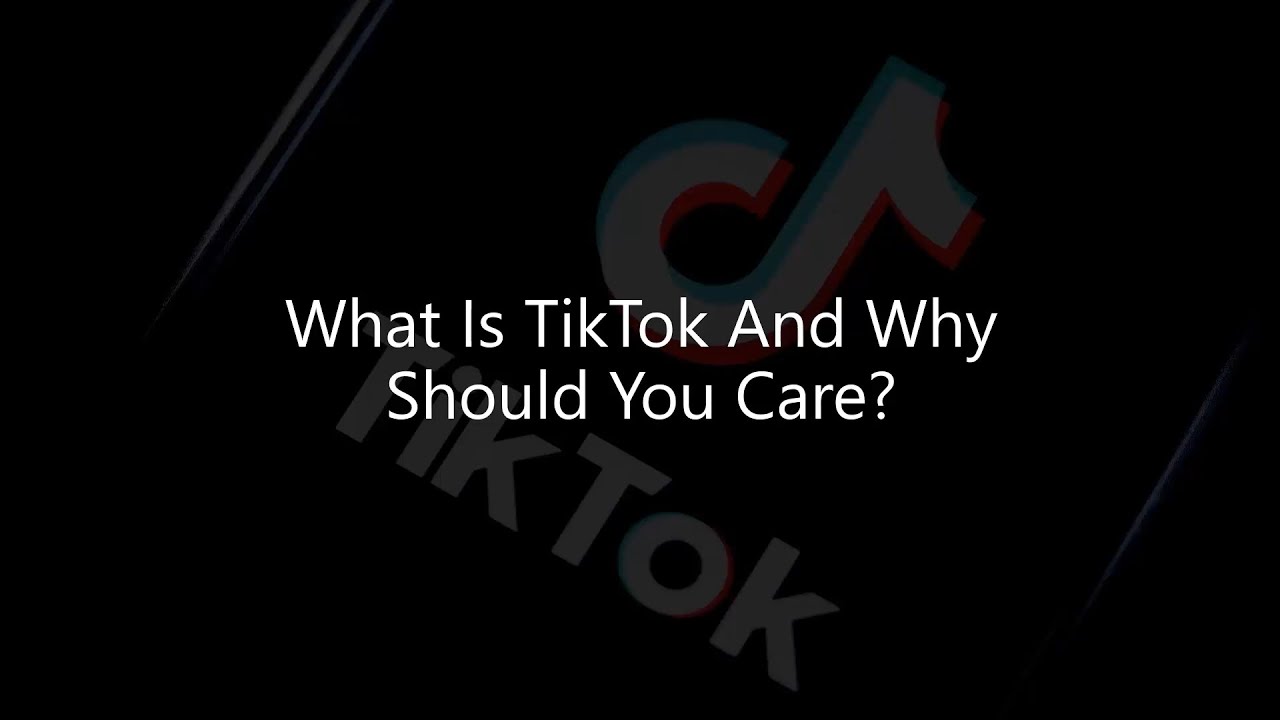The image appears to be a cover photo for an article. In the background, there is a blurred-out image of a smartphone displaying the TikTok app. Overlaying this background is the title of the article, written in white capitalized letters, "What Is TikTok and Why Should You Care?" The title stands out prominently against the grayed-out background photo, drawing attention to the subject matter of the article.